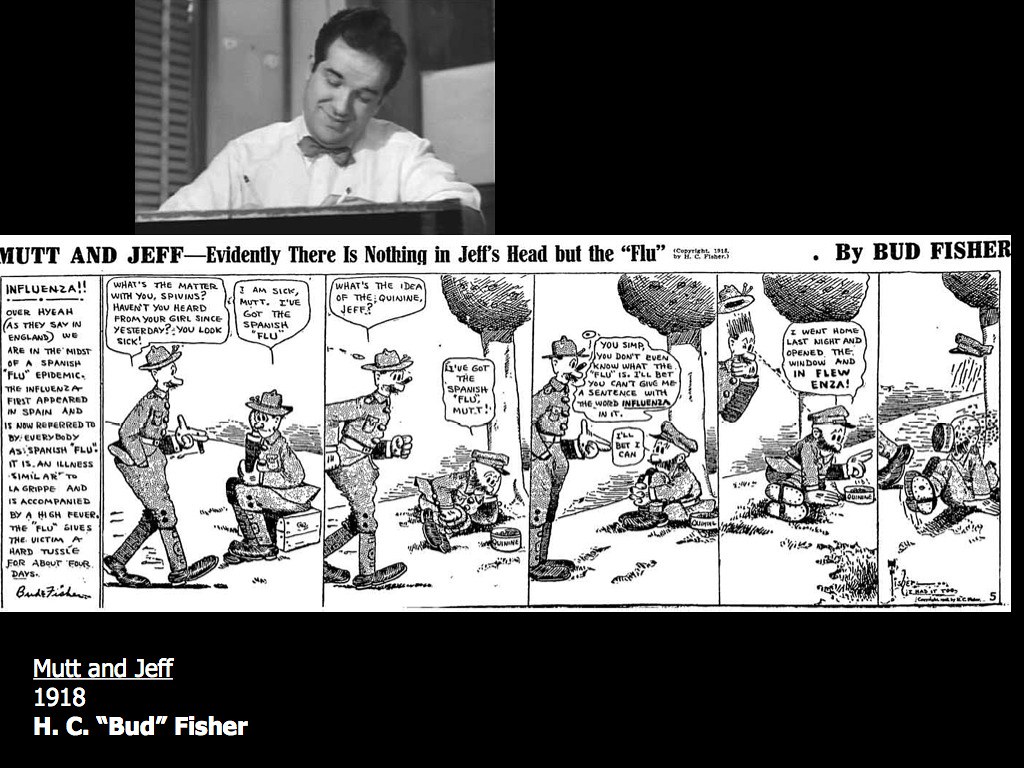The image features a classic cartoon titled "Mutt and Jeff" by H.C. Bud Fisher set against a predominantly black background. In the upper left corner, there is a black-and-white photograph of a man, presumably the artist Bud Fisher, wearing a suit and bow tie, evocative of the 1950s. Centered in the image is a black-and-white comic strip with different shades of gray, showcasing a humorous scene that implies Jeff has nothing in his head but the flu. The comic is labeled "Mutt and Jeff" in the bottom left corner along with the year "1918" and the artist's name, "H.C. Bud Fisher." The overall style and layout suggest this is an excerpt from a vintage newspaper comic strip.